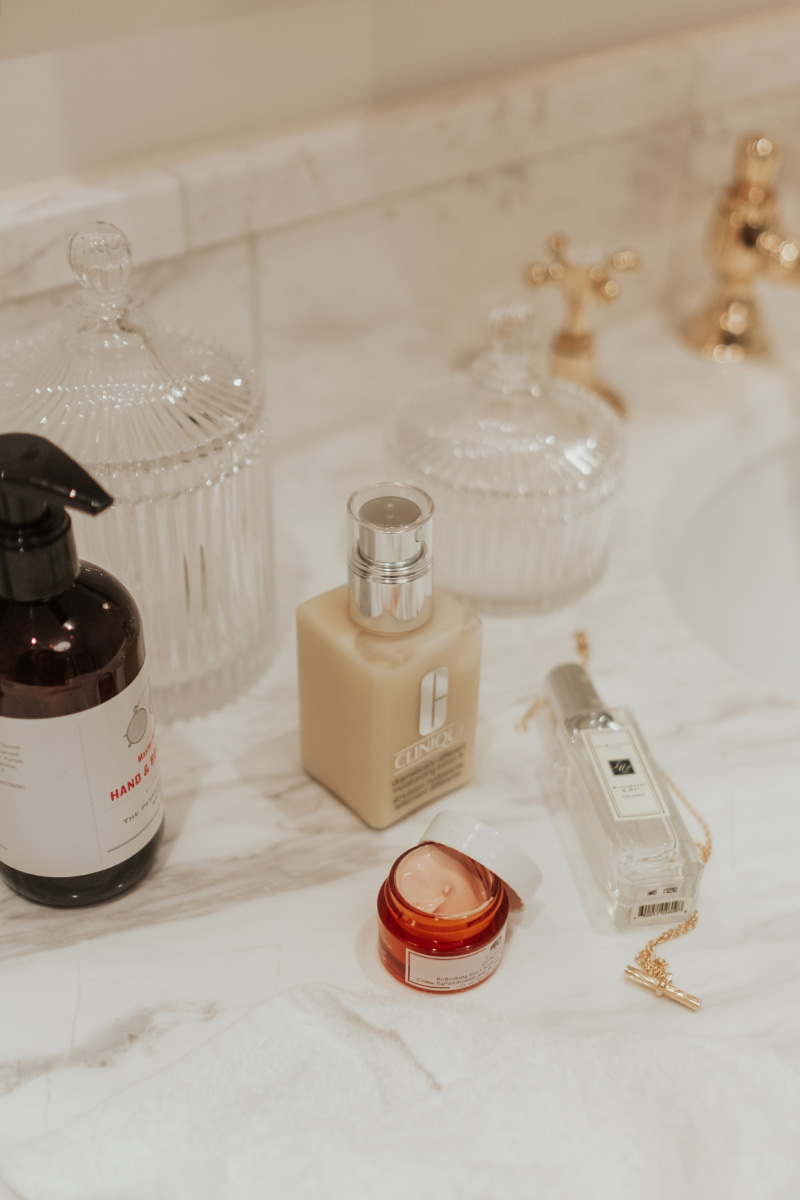The image depicts a well-organized bathroom counter made of elegant white marble with intricate gray swirls in a random, non-uniform pattern. At the center of this pristine counter, a variety of objects are neatly arranged:

1. **Brown Pump Container**: This container features a white label with red text reading "Hand in [unreadable]". The text is partially obscured, making the full label difficult to decipher.
   
2. **Two Clear Glass Containers**: One is significantly larger than the other, both boasting a sophisticated design, however, they are currently empty.
   
3. **Clinique Product Jar**: A square, upright jar which appears to be full, complete with its lid.

4. **Glass Rectangular Container**: A slim, clear container with a barcode sticker prominently visible on its bottom surface.

5. **Round Red Container**: This container, with a white cap propped open, reveals a tan cream inside.

Additionally, the sink boasts luxury with its gleaming gold handles, adding a touch of opulence to the overall aesthetic of the bathroom counter.